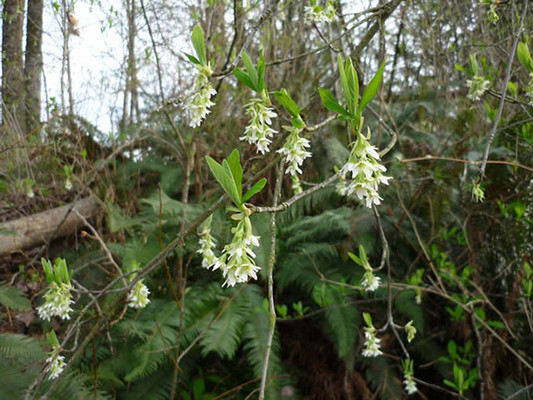This photograph captures a serene outdoor setting within a dense, wooded area. The focal point is a branch adorned with white flowers, reminiscent of snow bells, hanging downwards. These flowers, clustered with white petals, are juxtaposed against green leaves shaped like feathers, standing straight up. In the foreground, ferns lie on the ground, adding to the lush greenery. Behind the blooming branch, there is a forest-like backdrop with an array of bushes and tall trees. The trees have brownish-gray trunks, and one has fallen, laying horizontally on the ground to the left side of the image. The sky in the background appears overcast, casting a soft daylight glow across the scene. The photograph is devoid of people, animals, text, or any other objects, allowing the natural beauty of the flowers and the dense foliage to take center stage.